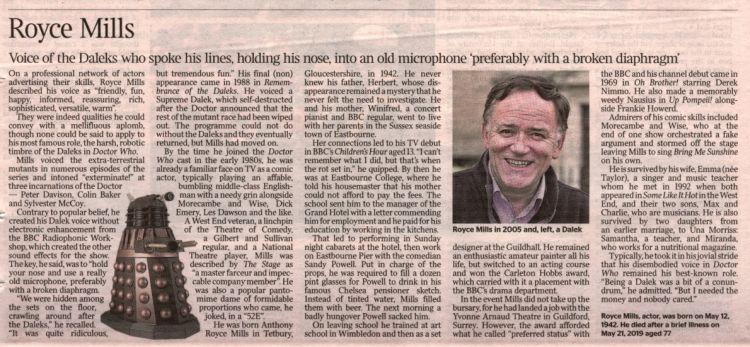Obituary Clipping for Royce Mills: Celebrated Voice of the Daleks

This image captures a newspaper obituary for Royce Mills, prominently featuring his name at the top in large script. Beneath his name, in slightly smaller script, the caption reads, "Voice of the Daleks who spoke his lines holding his nose into an old microphone, preferably with a broken diaphragm." This detail highlights his unique technique for voicing the infamous Daleks from the popular "Doctor Who" series.

The clipping includes two images. On the left, there is a photograph of a Dalek, the extraterrestrial robot from "Doctor Who." To the right, in a square frame, there is a portrait of Royce Mills. Mills, a white gentleman, is captured smiling warmly, dressed in a sweater and a button-down shirt. The caption under the portrait reads, "Royce Mills in 2005," situating the image in recent history.

The main body of the page consists of a detailed obituary chronicling Royce Mills' career and personal life. It closes with a succinct summary of his life: "Royce Mills, actor, was born on May 12, 1942. He died after a brief illness on May 21, 2009, age 77."